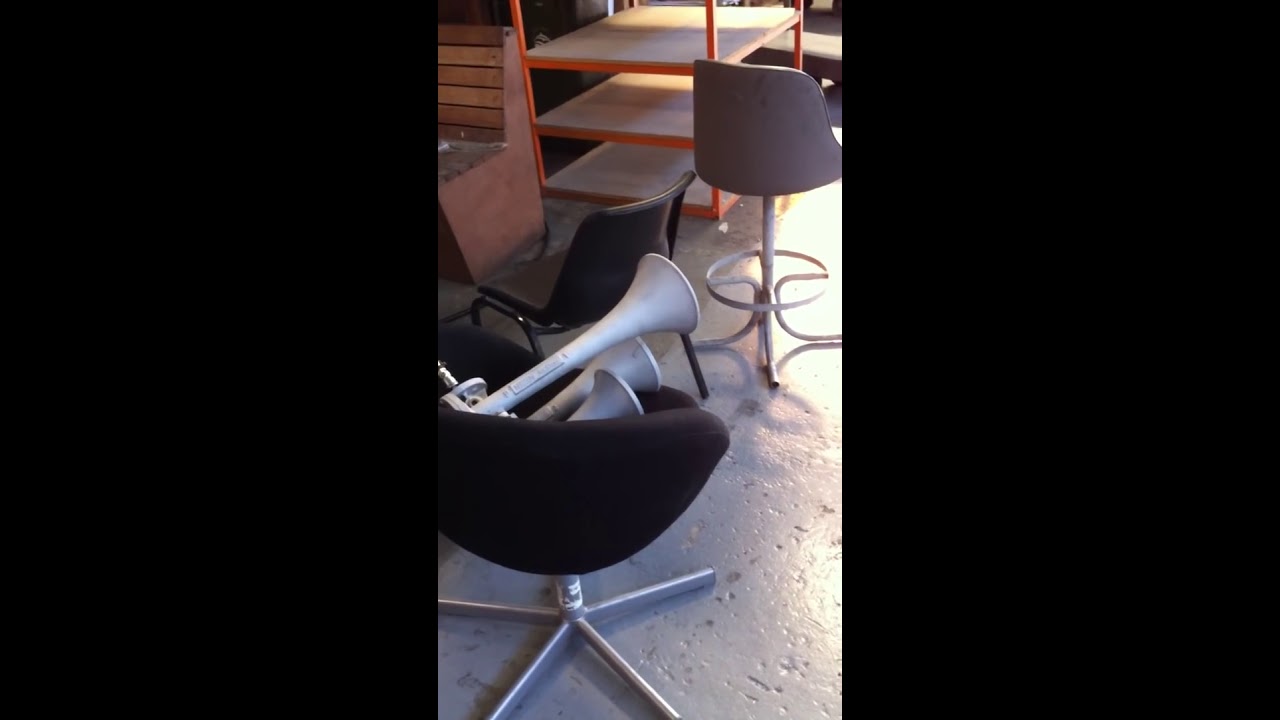This image features an arrangement of various chairs and furnishings set against a backdrop with distinctive black rectangular borders on either side. Dominating the center is a black, swiveling bucket chair affixed to a silver pole with a five-legged base for stabilization. This chair is facing away from the camera and contains a set of three white air horns. Surrounding it are other chairs, including one visible in the upper middle part of the image with a dark gray seat and a white pedestal base. There's also a glimpse of wooden bench seating in the top left corner, reminiscent of restaurant seating. Above, an orange-framed shelving unit with three light-colored wooden tiers, appears empty. The floor under the furniture looks to be made of white cement, contributing to the overall industrial workspace vibe of the scene. The image is captured vertically, providing a comprehensive view of this eclectic assortment of furniture and decor elements.